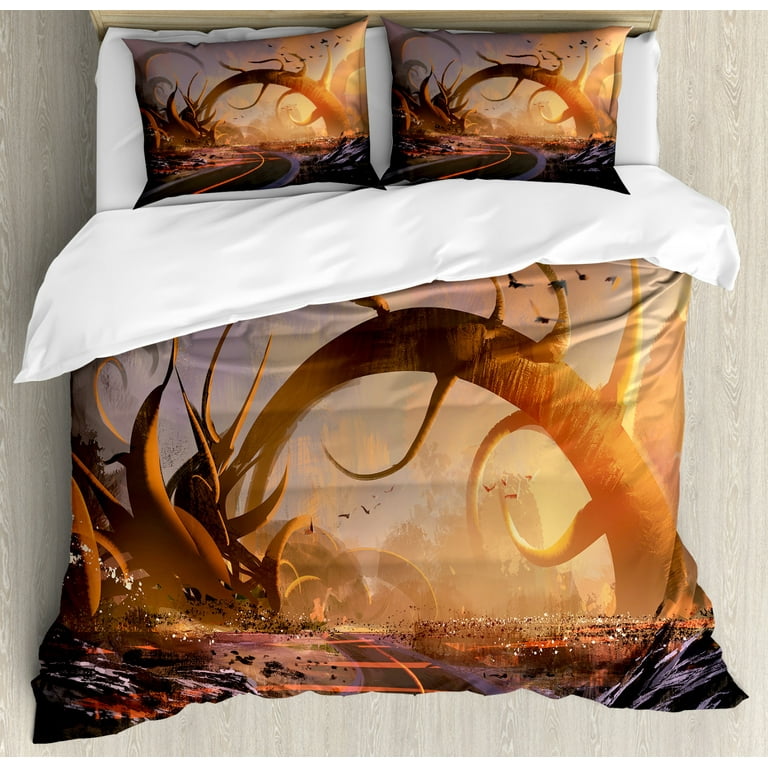This photograph, taken from an aerial perspective, captures a cozy full-size bed set against a light gray-beige wooden floor, highlighting the wood grain's intricate markings. The bed features a barely visible beige headboard at the top. The white sheets are partially pulled back to reveal two flat pillows, both adorned with a matching intense graphic print also found on the comforter. The bedding, featuring a puffy, pillow-like comforter, showcases a fantastical illustration of a large, bright orange and red tree with pointed tendrils extending from it. Birds fly amidst this scene, with abstract shapes resembling a road or train tracks weaving through the vibrant sunset-colored background. This detailed and imaginative design, capturing elements of a surreal fantasy landscape, suggests the image might be intended for a catalog or online shop. The layers of the bedspread and pillows add to the overall sense of comfort.